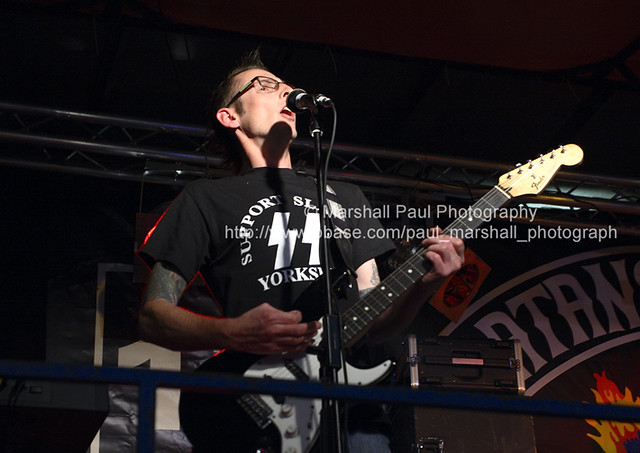In this image, a male singer with spiked hair and black-framed glasses is performing on stage. He is singing into a microphone on a stand, and is slightly to the left of the center, viewed from a slightly low angle. He is wearing a black t-shirt with white lettering, part of which reads "Support SL Yorkshire" and includes the initials "SS." His arms are marked with tattoos. The artist is playing a black and white guitar, and stands behind a blue railing that separates him from the audience.

The backdrop features a partially visible banner with the letters "T," "A," and "N" against a curved design, and a painted yellow and red flame on the right side of the image. Some musical equipment is visible behind him. The name "Marshall Paul Photography" is displayed across the middle of the image, along with a partially legible website URL beginning with "http://www.base.com/paul_marshall_photograph."